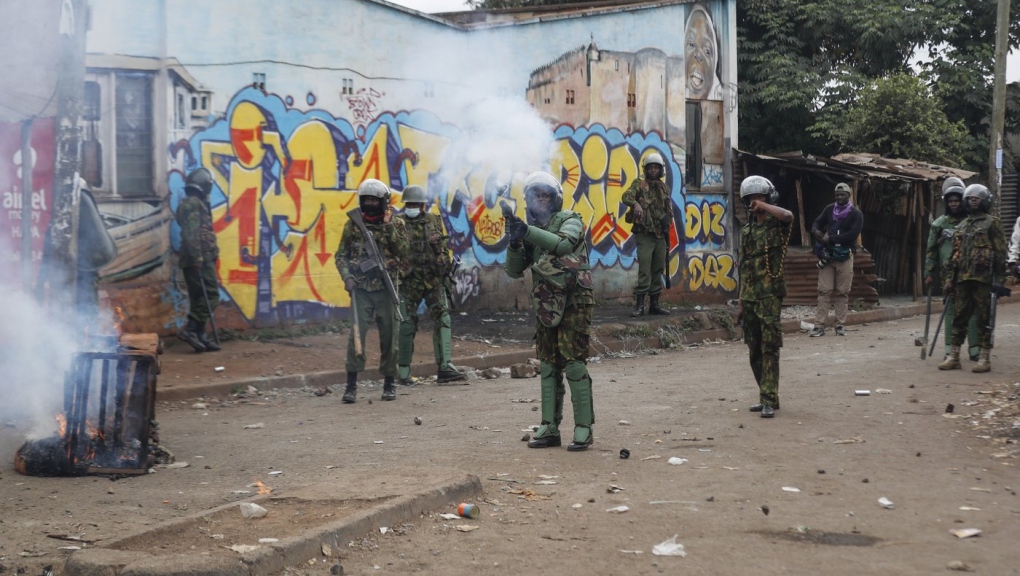The photograph captures a tense scene, likely set somewhere on the African continent, featuring nine soldiers in military attire complete with helmets, camouflage, and knee pads. The soldiers are dispersed across a street and all have their attention fixed on something behind and to the left of the camera's vantage point. Among the soldiers, one is seen firing a short gun that emits smoke, possibly a tear gas canister launcher aimed as a warning shot. Strewn across the ground are rocks, hinting at prior confrontations, while trash litters the area, adding to the chaotic atmosphere. To the left side of the image, a barrel is ablaze with flames and smoke billowing from it. 

The backdrop is dominated by a white wall adorned with bright, colorful graffiti featuring yellow and red writing bordered with blue, and an intricate mural depicting a tall building and a child of color, whose expression is ambiguous, either smiling or grimacing. A lone individual, possibly a journalist or a passerby, stands apart from the soldiers, equipped with a camera, observing the unfolding scene. The vibrant yet damaged environment underscores the tension captured in this vivid, color photograph.